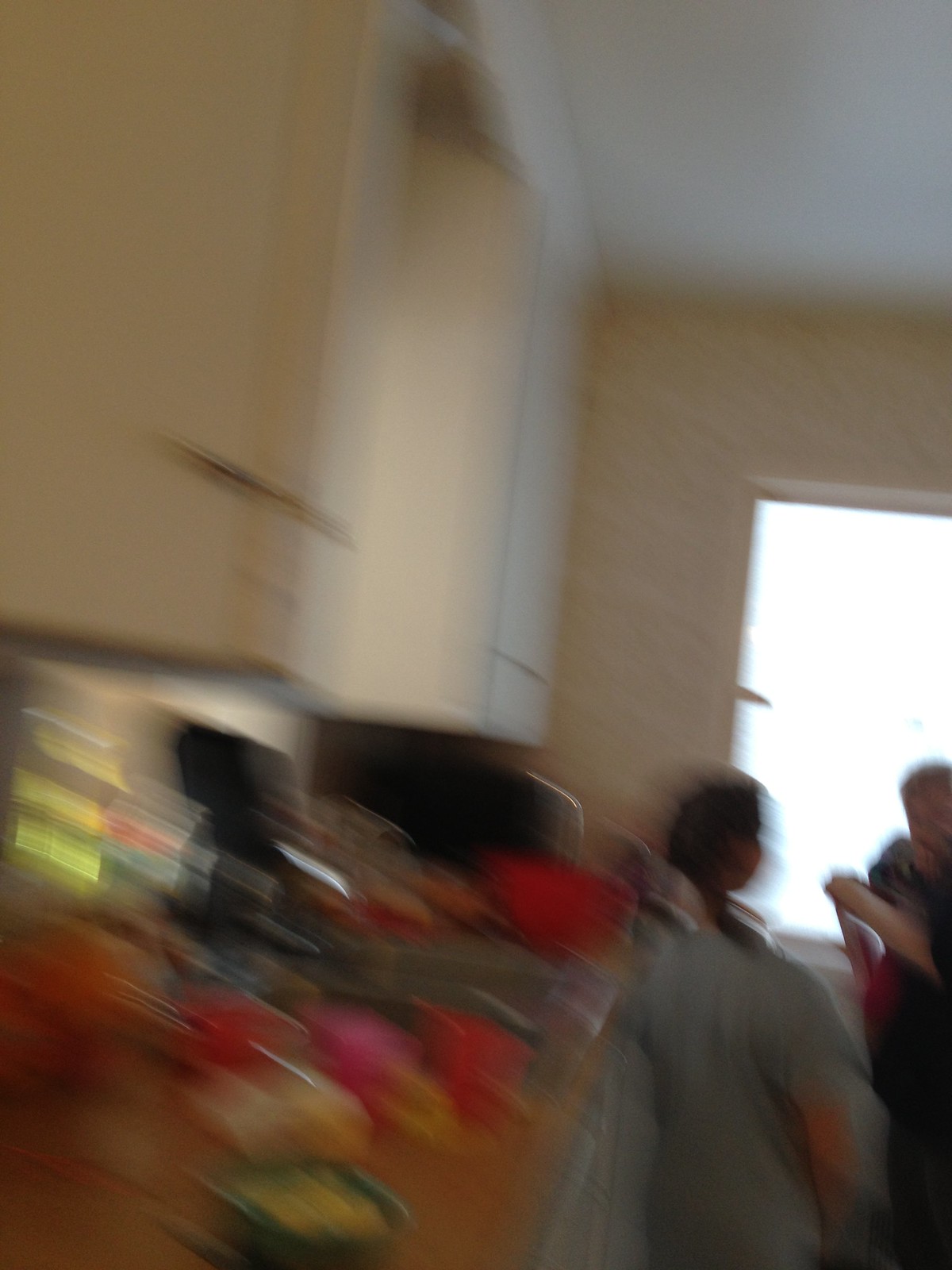This vibrant color photograph captures a cozy indoor gathering at someone's home. The scene is slightly obscured by a blur, lending an air of intimacy and nostalgia. In the bottom right corner, partly visible, is a table situated in front of a window, where a few guests are seated, engaged in conversation. On the left side of the image, a counter laden with various items gives a glimpse into the everyday life and perhaps preparations for the get-together. Above the counter, kitchen cupboards add to the homely atmosphere. The overall blur of the photo suggests a candid moment, preserving the warmth and conviviality of the occasion.